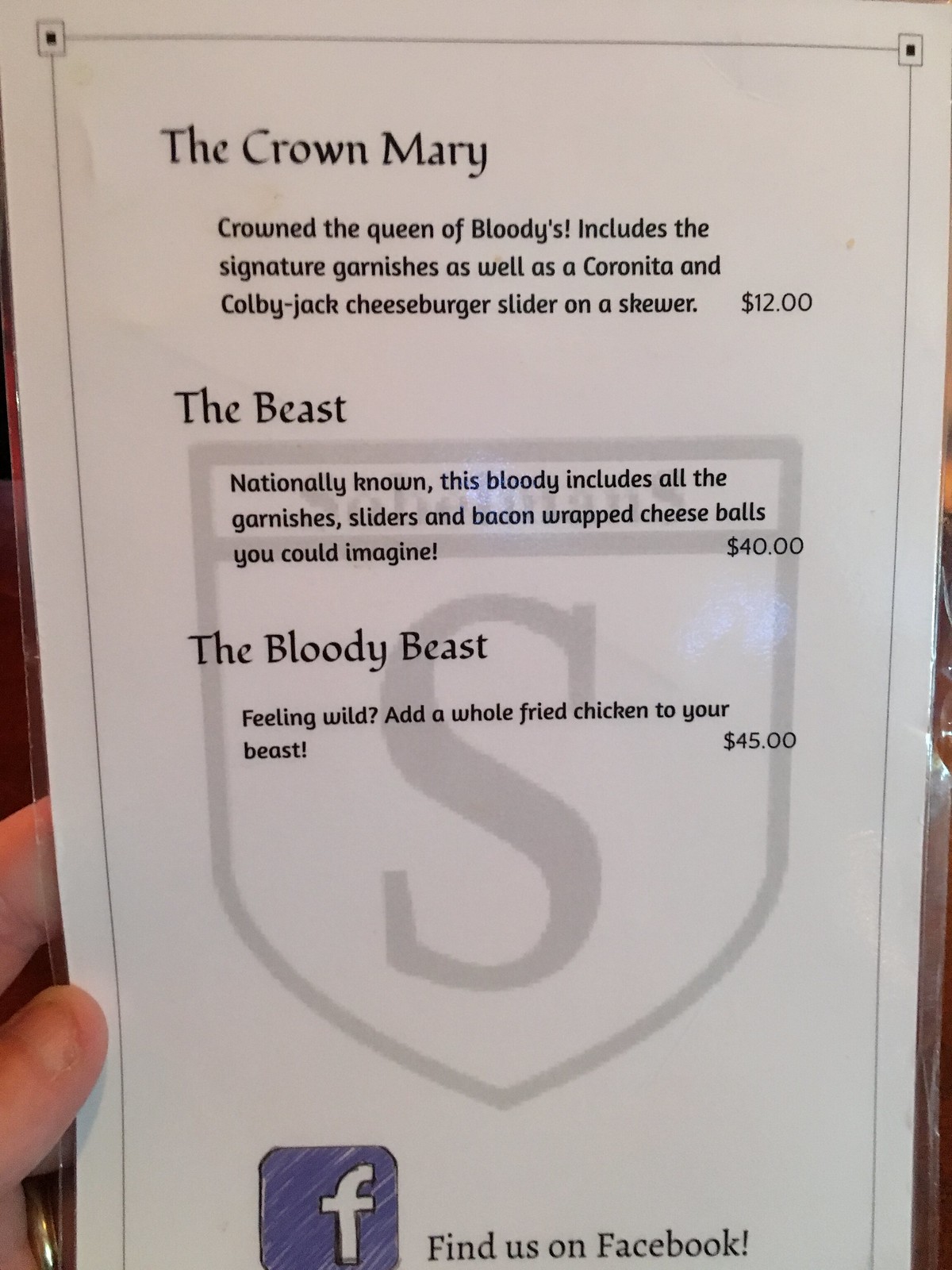In this detailed portrait-style image, a menu is prominently displayed, occupying most of the frame, presumably taken by a camera. On the left edge of the image, a small portion of a thumb is visible on the front side of the menu, with the index finger positioned behind it, suggesting someone holding it.

At the top of the menu, bold black text reads, "The Crown Mary," followed by a tagline in smaller black font: "Crowned the Queen of Bloodies." This section describes a unique offering that includes signature garnishes along with a Coronita beer and a Colby Jack cheeseburger slider on a skewer, priced at $12.

Below this, another item is featured: "The Beast," described as "nationally known." This extravagant bloody drink includes a plethora of garnishes, various sliders, and bacon-wrapped cheese balls, listed for $40.

The next item, "The Bloody Beast," ups the ante by suggesting the addition of a whole fried chicken to "The Beast" for a total price of $45, appealing to those feeling particularly adventurous.

Subtly visible in the background of the menu is a faded grey shield with the letter 'S' inside, adding a touch of design to the otherwise straightforward layout.

At the very bottom of the white menu, a hand-drawn Facebook logo accompanied by the text "Find us on Facebook" invites patrons to connect on social media. This information is placed neatly at the bottom of the image, closing off the portrayal of the menu.

Overall, the image vividly captures the elaborate and creatively named offerings of the establishment, giving a clear and enticing overview of their featured bloody drinks.